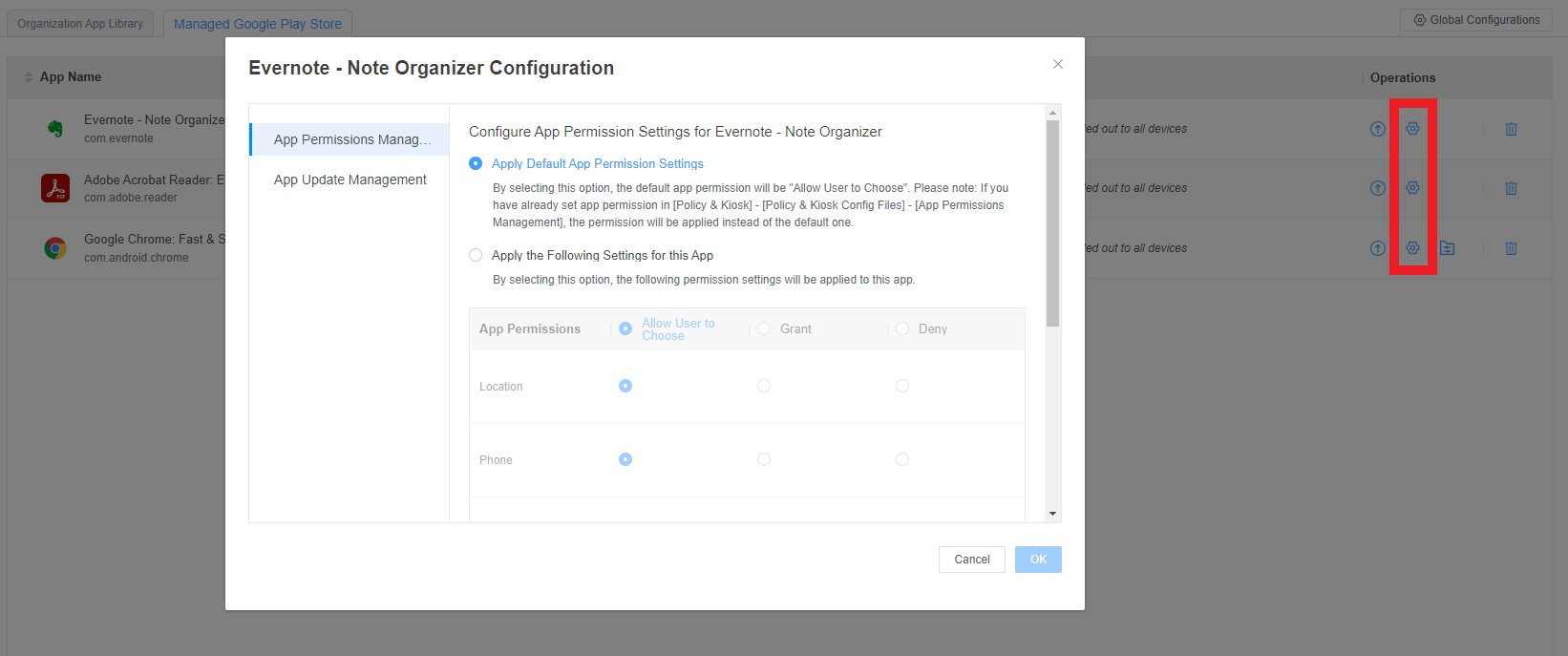The image depicts a user interface screen with a predominantly dark gray background. On the right side of this background, a set of dots is highlighted by a thin, red vertical rectangle.

In the center of the image, a white rectangular box is present. This box contains several lines of text. At the top of this white box, it reads "Evernote - Note Organizer Configuration."

Beneath this line, there is some whitespace followed by a light gray-bordered rectangle. Inside this rectangle, there is a blue button labeled "App Permissions Manage," where the word "Manage" is partially obscured, only showing as "M-A-N-A-G."

Further down, on the white background, you see the text "App Update Management" with additional explanatory text slightly to the right: "Configure app permission settings for Evernote - Note Organizer." Below this description, in blue text, it says, "Apply default age permission settings."

Towards the bottom, the text becomes too small to decipher fully except for a section that includes a small graph or table detailing "App Permissions" categorized under "Location" and possibly "Home."